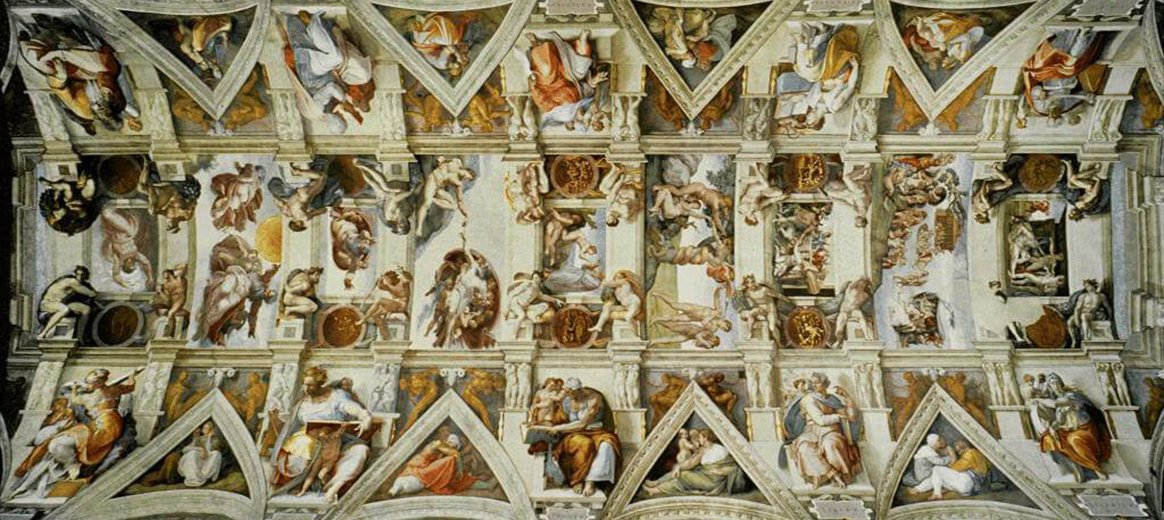The image captures a richly detailed and intricate ceiling, most likely from a church or cathedral, reminiscent of the famous Sistine Chapel. The ceiling is curved, and the perspective is from below, looking up at the stunning scenes. The artwork is composed of multiple sections, including rectangular and triangular segments, detailing various biblical events and figures, such as angels and historical human interactions. The color palette is warm and antiquated, featuring hues of red, brown, cream, green, and dark blue, giving it a timeless and historic appearance. The vivid and well-preserved images are intricate and carefully arranged, reflecting the depth of classical religious art.